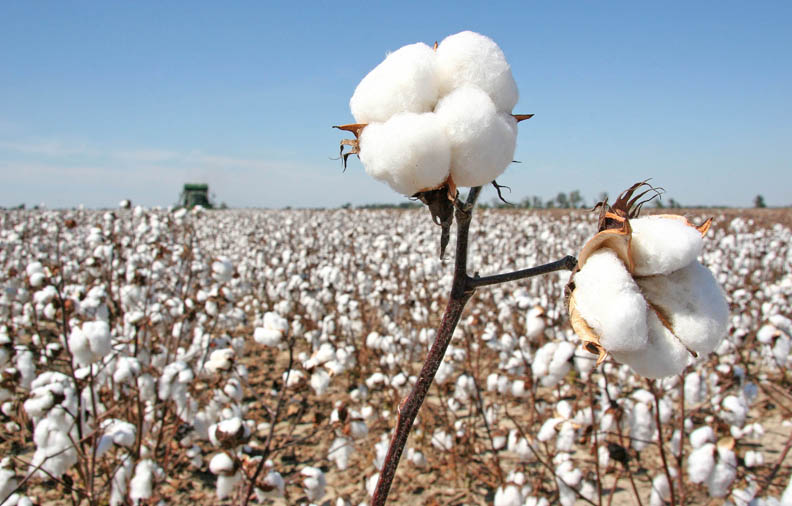The image depicts a vast cotton field in full bloom under a bright, blue sky with only a few wispy clouds overhead. Dominating the foreground, a single cotton plant stands out in sharp focus, its brown stem adorned with two primary stalks, each boasting four white cotton bulbs. The cotton field stretches out behind this focal plant, with numerous tall cotton stalks ready for harvest, their abundant bulbs slightly bending. In the distant background, a grey harvesting truck can be seen, suggesting the field's imminent collection. Beyond the endless sea of cotton, small trees mark the horizon, indicating the next field, which appears already harvested. This picturesque scene captures both the expansive beauty of the cotton field and the intricate detail of a single, blooming cotton plant.